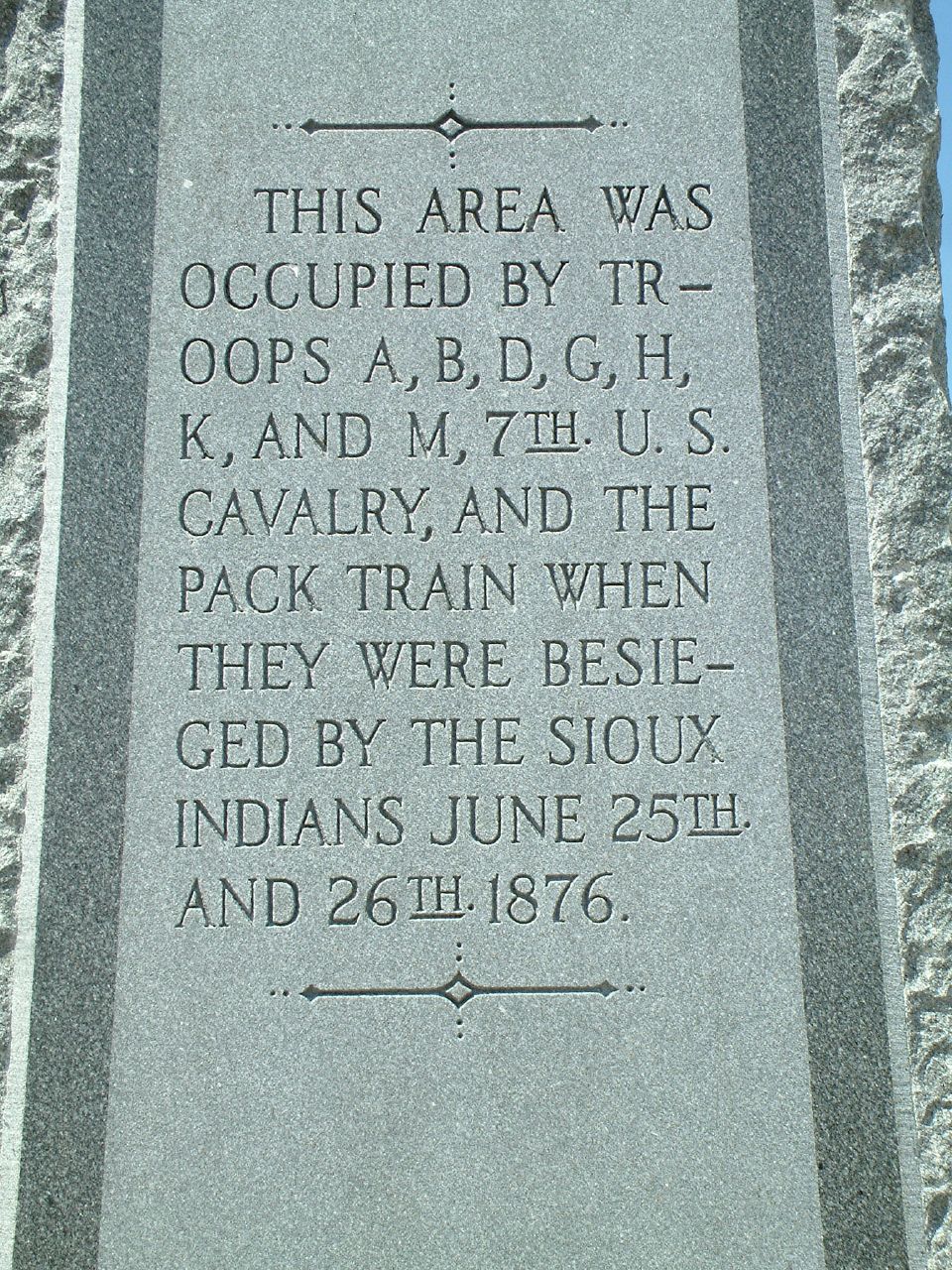The image depicts a close-up of a monument dedicated to members of the 7th U.S. Cavalry. The monument is made of rough, ridged granite on the sides, with a smooth, well-maintained central area where the engraving is found. The inscription reads: "This area was occupied by troops A, B, D, G, H, K, and M, 7th U.S. Cavalry and the pack train when they were besieged by the Sioux Indians, June 25th and 26th, 1876." The text is in all capital letters, deeply carved into the stone. Above and below the inscription, there are decorative lines with a diamond shape in the center and dots at the ends, aligned both vertically and horizontally. The backdrop visible in the image includes a clear blue sky, enhancing the solemnity and clarity of this historical monument.